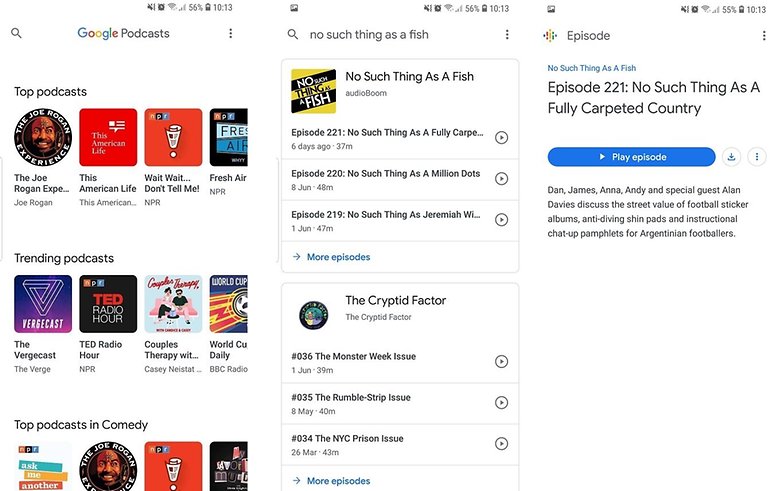The image depicts a web page for Google Podcasts. At the top left corner, the title "Google Podcasts" is prominently displayed. Below the title, there is a section showcasing the "Top Podcasts" arranged from left to right. The featured podcasts include "The Joe Rogan Experience," "The American Lie," "Wait Wait... Don't Tell Me!" and "Fresh Air."

Following this, there is a section labeled "Trending Podcasts," which highlights "The Vergecast," "TED Radio Hour," "Couples Therapy," and "World Cup Daily."

Another section is dedicated to "Top Podcasts in Comedy," listing "Ask Me Another," "The Joe Rogan Experience," "Wait Wait... Don't Tell Me!" and an additional podcast where the title and image details are not clearly visible.

In the second column on the page, the podcast "No Such Thing As A Fish" is featured, displaying episodes 221, 220, and 219. Additionally, "The Cryptid Factor" is shown with episodes 36, 35, and 34.

The last column on the right focuses on episode 221 of "No Such Thing As A Fish," titled "No Such Thing As A Full Carpeted Country." There is a "Play Episode" button, followed by a descriptive paragraph mentioning that hosts Dan, James, Anna, and Andy, along with special guest Alan Davies, discuss topics such as the street value of football sticker albums, anti-diving shin pads, and instructional chat-up pamphlets for Argentinian footballers.